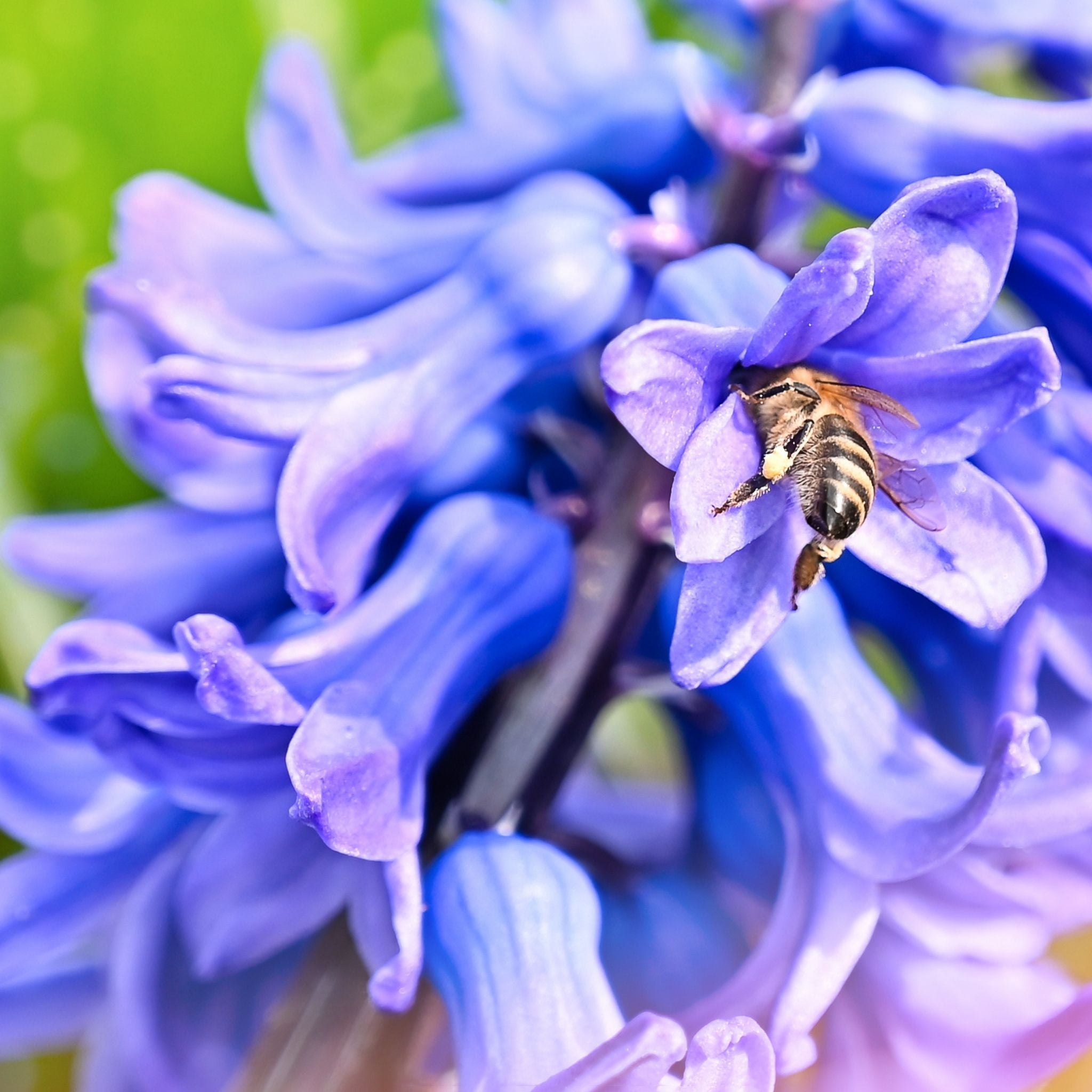This highly detailed color photograph, taken outdoors in portrait orientation, features a stunning close-up of a cluster of beautiful purple Hyacinth flowers. The primary focal point is a honeybee, situated slightly to the right of center, its head delved deep into one of the tubular, bell-shaped hyacinth blossoms. The bee's yellow and black striped abdomen, distinguishable by its fuzzy yellow hairs, is prominently visible along with three of its segmented legs. One leg is adorned with a cluster of yellow pollen. The bee's transparent, light brown wings are fanned out from its back, adding to the intricate details of the scene.

The hyacinth flower at the center-left is fully in focus, showcasing seven vivid purple petals that indicate its distinctive species. This flower, like the others in the cluster, extends from a light gray stem that diagonally bisects the photo from the bottom left to the top right. The background is a blur of green, suggesting a grassy field or similar outdoor setting, reinforcing the image’s realistic representation of nature.